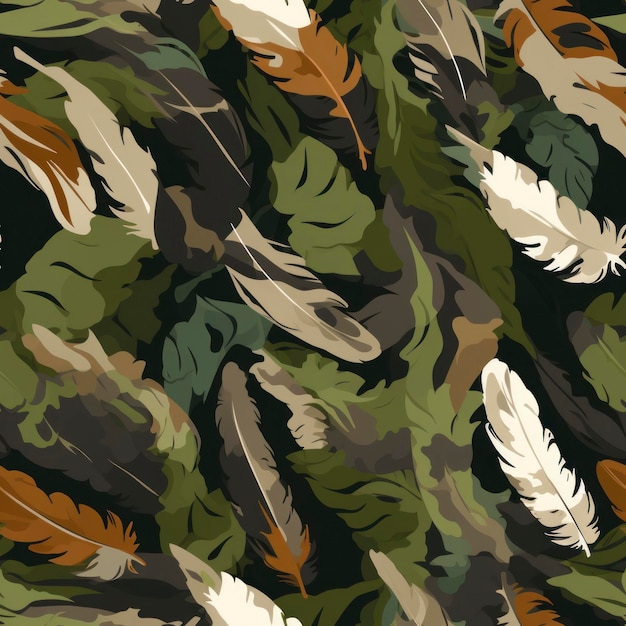This digital illustration depicts an abstract arrangement of feathers and leaves set against a dark black background, evoking a camouflage pattern through its earthy color palette. The feathers are rendered in various shades of beige, brown, rust, green, and white, creating a harmonious transition of natural tones. Key details include a beige feather with a striking white stripe, a dark brown and green feather, and a rusty feather intertwined with beige. Muted greens and beiges dominate the center, while two distinct tan and white feathers stand out on the far right. Interspersed among the feathers are different types of leaves in grey and multiple shades of green, adding to the depth and complexity of the image. The intricate composition and the blending of colors suggest a sophisticated digital artwork suitable for use as a computer background.